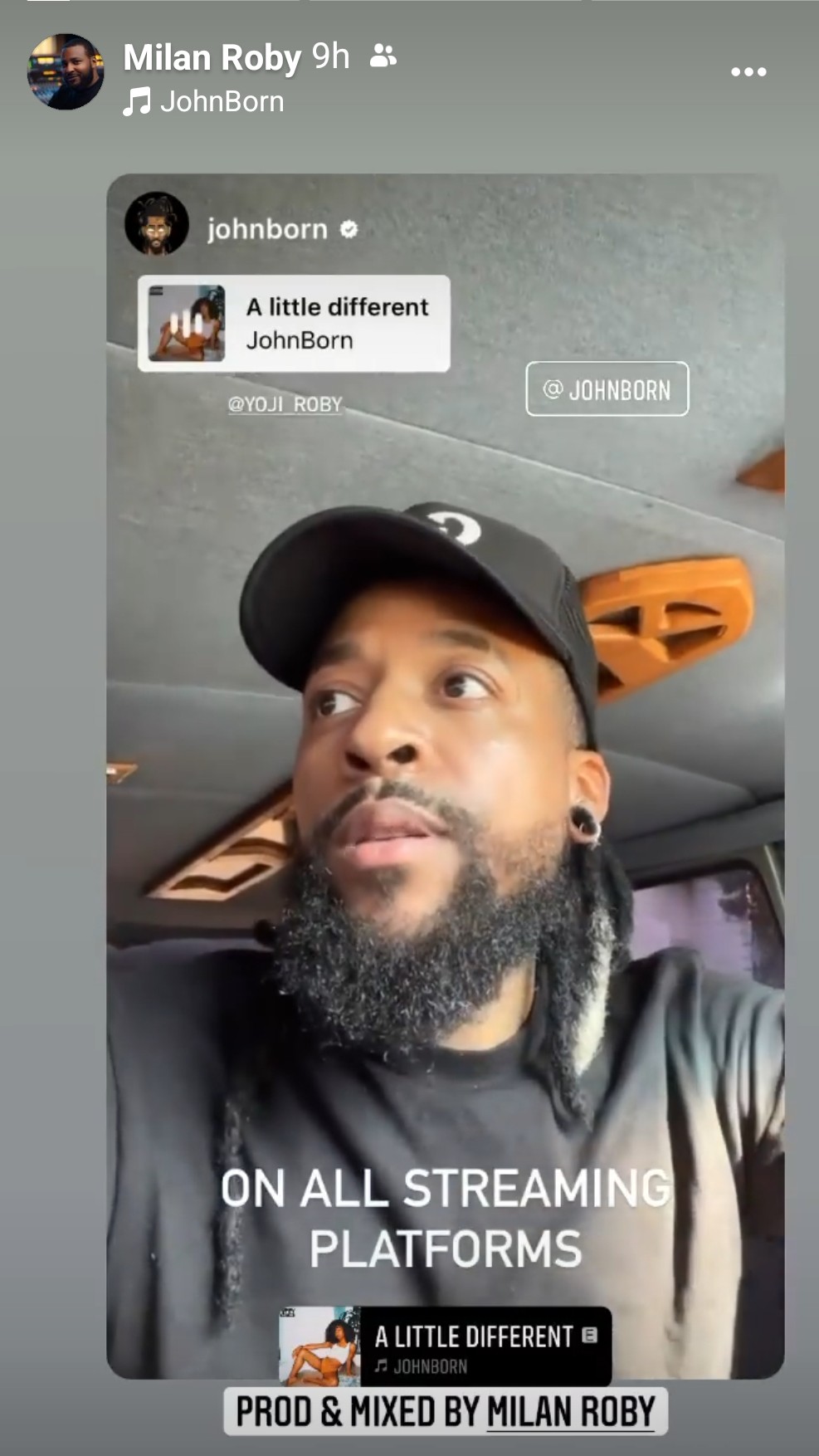Here's a detailed and cleaned-up caption for the image:

---

In a social media screenshot, Milan Roby's post is displayed prominently at the top. His profile features a picture of him, and his username is clearly shown as "Milan Roby" (R-O-B-Y). Accompanying his post is a music note emoji and a message highlighting John Bourne's latest work. Milan has shared a repost of John Bourne's new release titled "A Little Different." Below this message is a vivid picture of John Bourne, showcasing him as an African man with gauged ears, a well-groomed beard, mustache, and dreadlocks. He is seen wearing a ball cap and a gray T-shirt. The promotional art in the post highlights that "A Little Different" is available on all streaming platforms and notes that the track is produced and mixed by Milan Roby. This post signifies Milan Roby's role in the production and mixing of John Bourne's latest release.